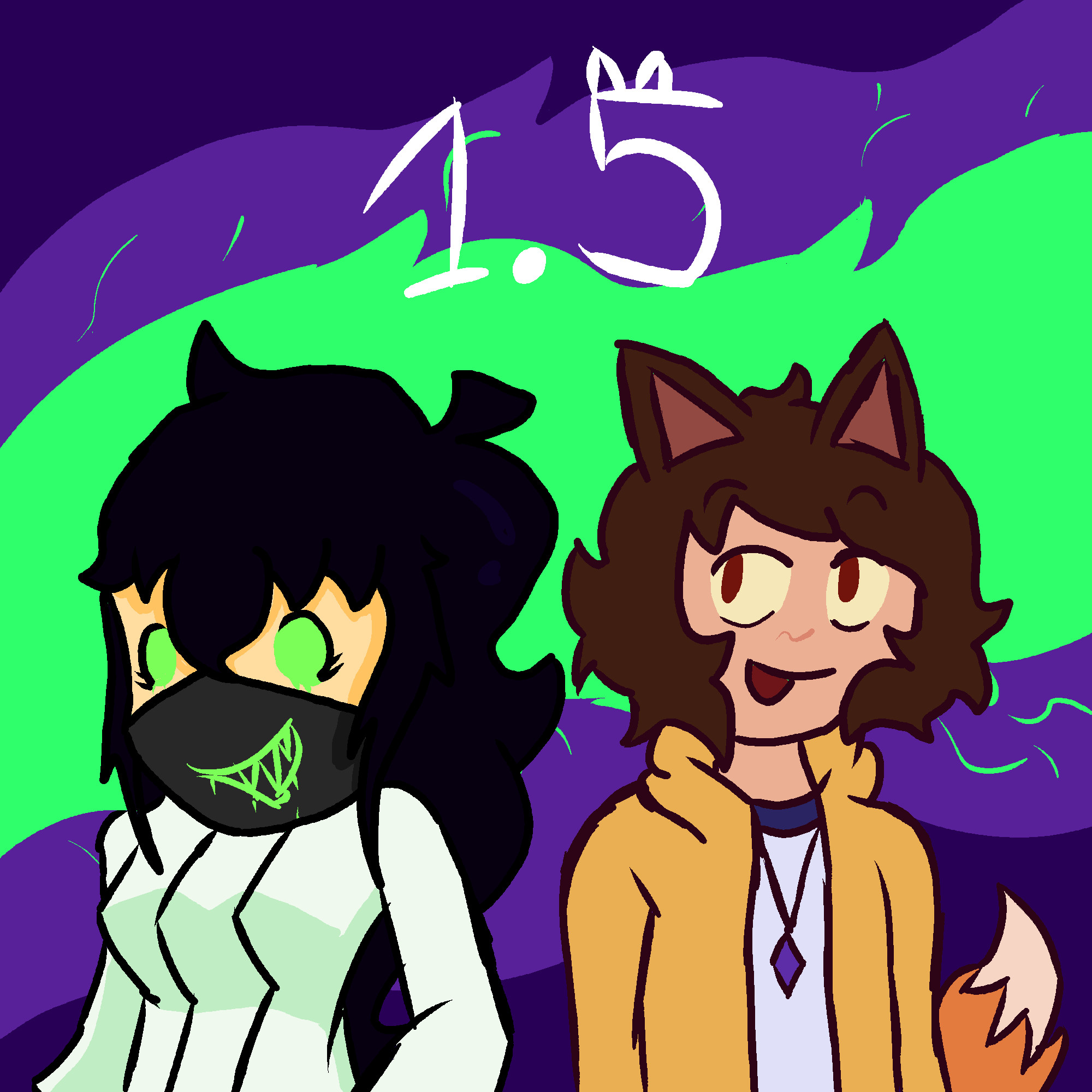The image is a large, square, computer-animated illustration featuring two characters, possibly cartoon figures or original creations. The background displays a sequence of wavy patterns: dark blue at the upper left corner, transitioning to a purplish-blue, bright green in the middle, and back to purplish-blue and navy at the bottom. At the top, the hand-drawn number "1.5" in white, with the "5" embellished with bunny ears, is prominently featured.

On the left stands a female character with black hair and neon green eyes, masked with a neon green design depicting a mouth. She wears a white long-sleeve top adorned with vertical lines and a touch of lime green. The character on the right, likely male, sports bunny ears on brown hair, a tan jacket with a chain and a diamond-shaped pendant, and a white t-shirt underneath. He has a friendly smile and appears to be interacting with the female character. Additionally, he might feature a tail with orange and cream colors, visible on the right side. The overall scene is vibrant and engaging, framed by a dynamic and colorful background.